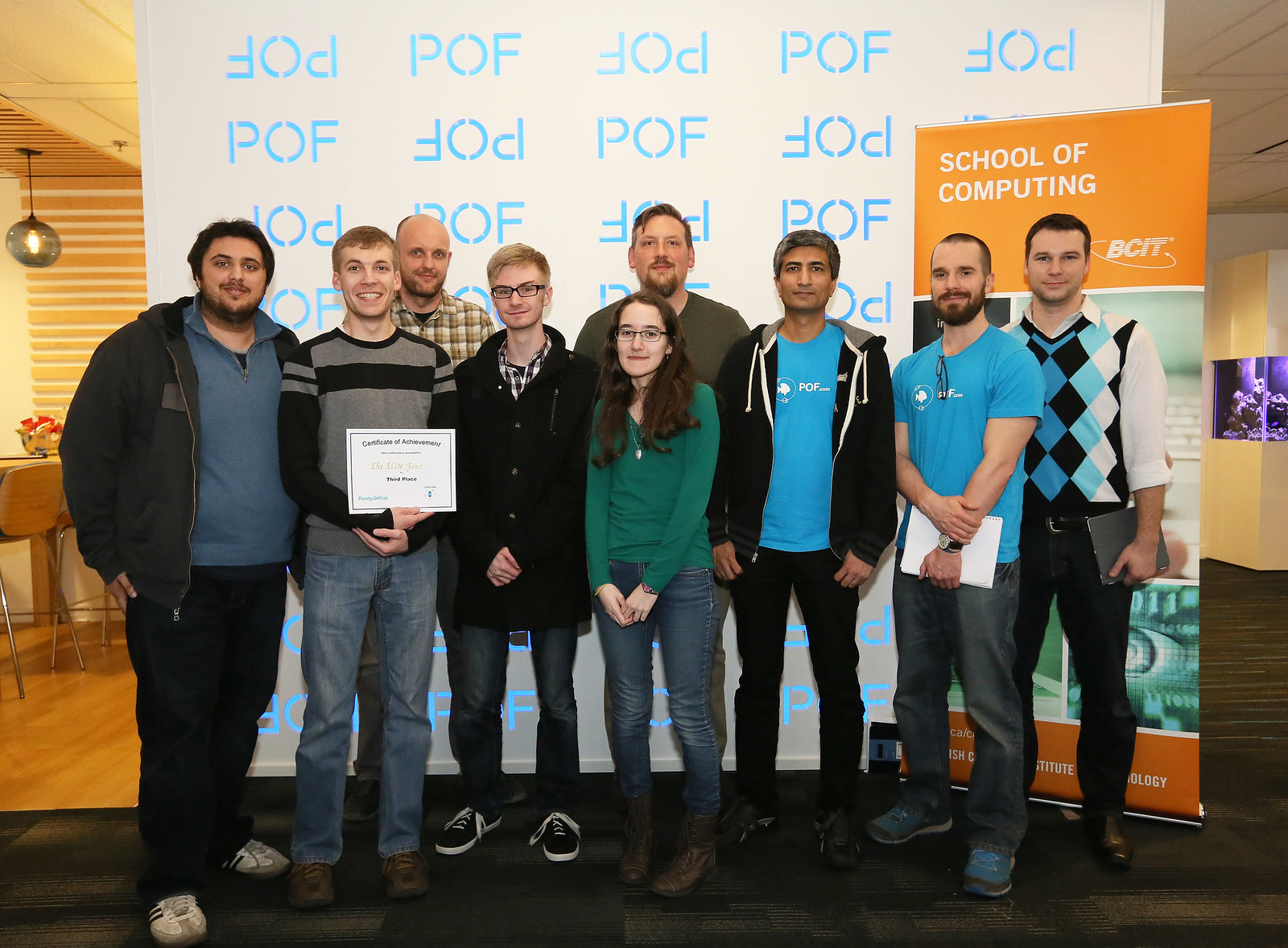In the image, a group of nine young adults, including eight men and one woman, are posing together, likely at a conference or school event. The individuals are dressed in casual attire, with long-sleeved tops, t-shirts, jeans, and sneakers. A young man on the far left is proudly holding up a white "Certificate of Achievement," indicating he won something, possibly third place. The backdrop features a patterned white wall with the letters "P-O-F" in various orientations, some upside down and backward. Prominently displayed on the right side of the image is an orange banner that reads "School of Computing," suggesting an academic or professional setting within a school environment. The scene also includes subtle details like a possible kitchen area to the left and a fish tank on the right, enhancing the casual, yet scholastic atmosphere.